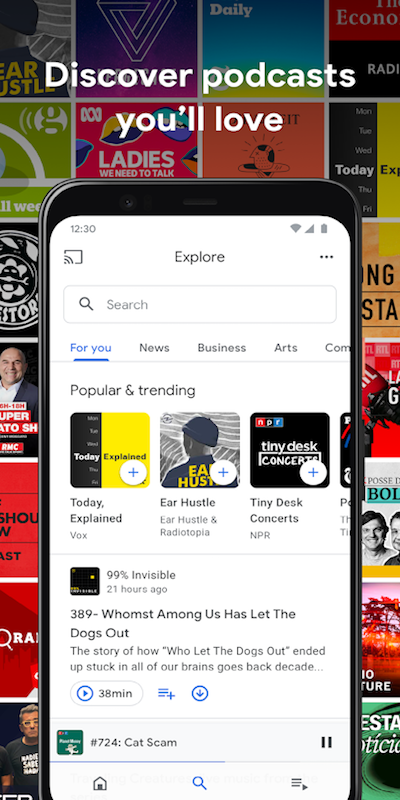The image features a vibrant and dynamic background filled with various titles of TV shows and movies, none of which are immediately recognizable. Dominating the top portion, in bold white letters, is the phrase "Discover Podcasts You'll Love." Central to the image, a smartphone is prominently displayed with a sleek black border and a white screen, showing the time as 12:30 and icons for Wi-Fi, signal bars, and battery status. Below the phone, large text encourages viewers to "Explore."

Further down, a search bar adorned with a magnifying glass icon invites users to find content. Directly beneath, several categories are listed for exploration: "For You," "News," "Business," "Arts," and "COM." Following this, the "Popular and Trending" section is showcased, featuring three podcast thumbnails from left to right.

The first thumbnail promotes "Today, Explained" by Vox, followed by "Ear Hustle" produced in conjunction with Radiotopia. The third thumbnail highlights "Tiny Desk Concerts" by NPR. Below these thumbnails, detailed captions provide additional context:
1. "99% Invisible - 21 hours ago: 389 'Whomst Among Us Has Let the Dogs Out' - A story of how 'Who Let the Dogs Out' became a decades-long earworm."
2. "38 minutes ago: 'Cat Scam.'"

The overall vibe of the image is geared towards enticing viewers to delve into a world of podcasts, expertly curated to cater to a wide array of interests.